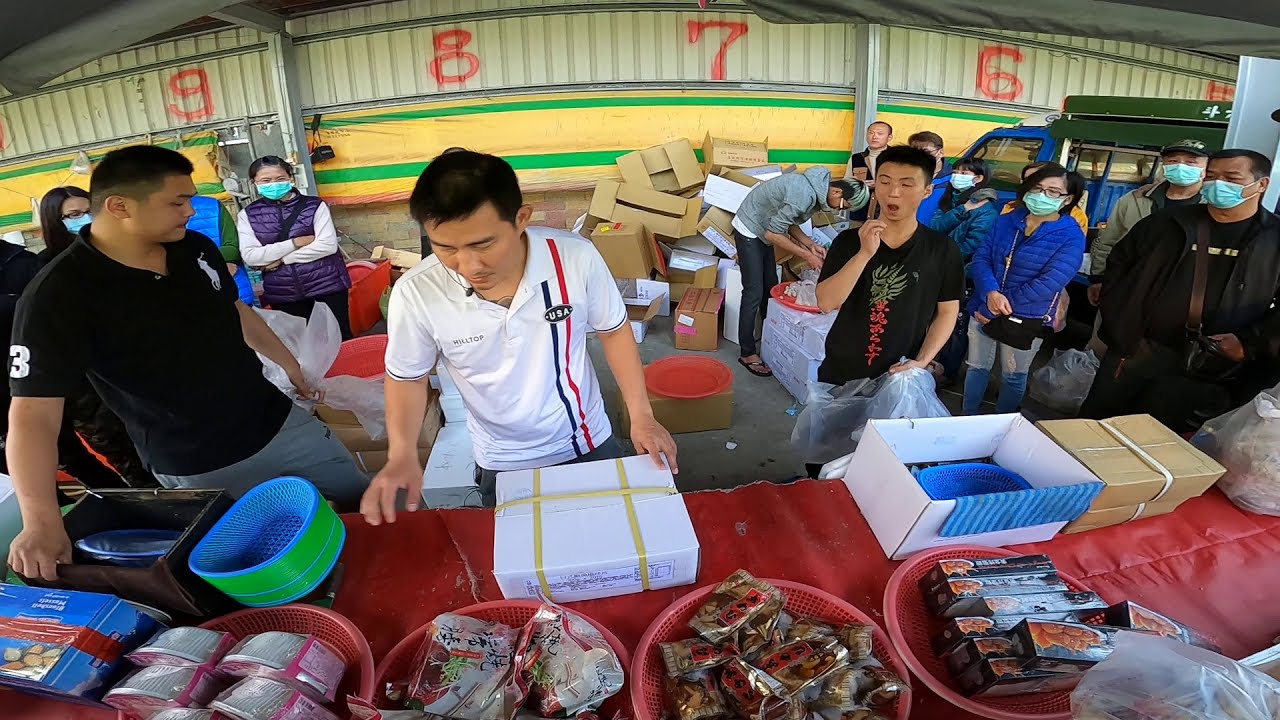This is a horizontally aligned, rectangular photo capturing a busy outdoor scene at what appears to be a food distribution event, possibly in an open-air market or under an outdoor warehouse. Centered in the image is a long table draped with a red tablecloth. Atop the table are various food containers, including large red bowls filled with packets of food items, as well as green and blue oval-shaped food baskets. A white box is visible in the middle of the table, flanked by an open cardboard box and another closed one.

In the foreground, three men are lined up at the table. The man in the middle is dressed in a white polo shirt and seems to be interacting with the white box, while the men flanking him wear black shirts. Positioned behind this main trio, and to the right, is a larger group of people, some wearing paper masks over their faces. A similar group is seen to the left, also wearing masks. In the background, the scene is framed by a yellow wall with large, red numbers painted sequentially from nine to six. Below this wall, a striped pattern of yellow and green is visible. Cardboard boxes are haphazardly stacked along the wall. To the far right of the image, partially cut off, is a blue and green truck. The photo provides a vivid, detailed snapshot of the orderly yet bustling atmosphere of the event.